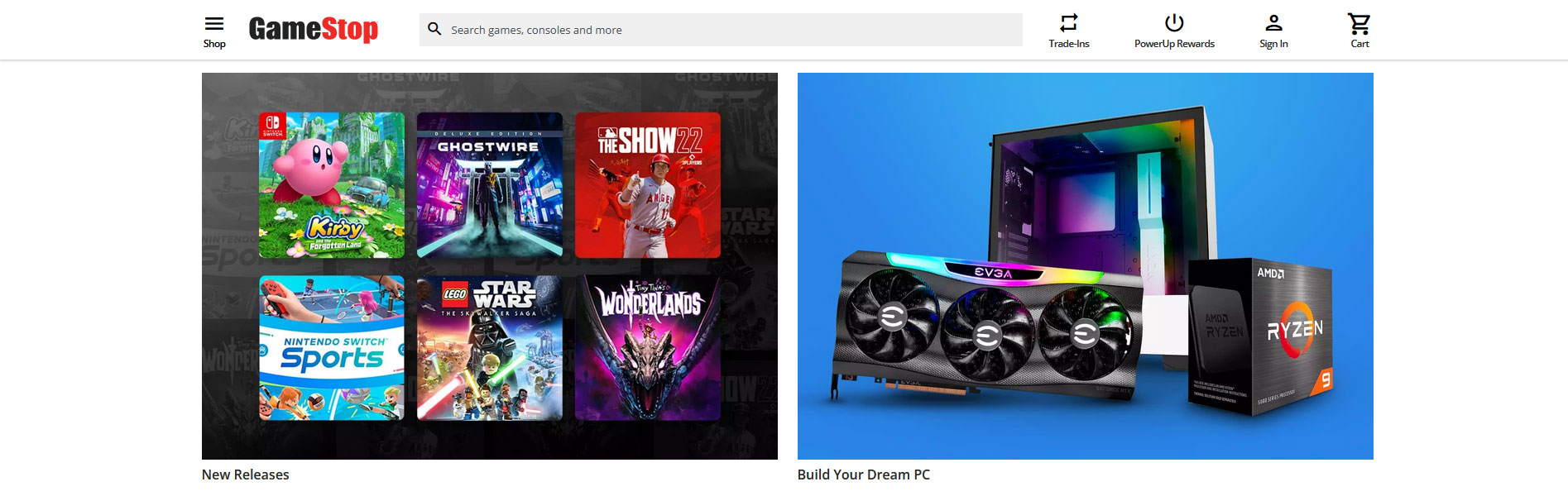This is a detailed screenshot of the GameStop website homepage. In the upper left-hand corner, the GameStop logo is prominently displayed. To the left of the logo, there is a "Shop" label indicating a menu available for browsing various categories and products.

Adjacent to the right of the GameStop logo, there is a search bar with a placeholder text that reads, "Search games, consoles, and more". This allows users to quickly find specific items they are looking for. Following the search bar to the right, there are several button options, including "Trade-Ins", "PowerUp Rewards", "Sign In", and "Cart".

Beneath this main navigation area, the webpage is divided into two primary sections. The left section is dedicated to "New Releases" and showcases six featured game titles. The first game displayed is "Kirby", followed by "Nintendo Switch Sports", "Lego Star Wars", "Tiny Tina's Wonderlands", "MLB The Show", and "Ghostwire: Tokyo".

On the right side, there is a section labeled "Build Your Dream PC". This section includes an image featuring various computer components. The image is somewhat ambiguous, but it includes a prominently featured black box labeled "RYZEN" in white text with a striking red circle emblem, indicating it's likely a processor from AMD’s popular Ryzen series.

Through the detailed layout, users can easily navigate the GameStop website to explore new game releases and find essential components for building their personalized PC setups.